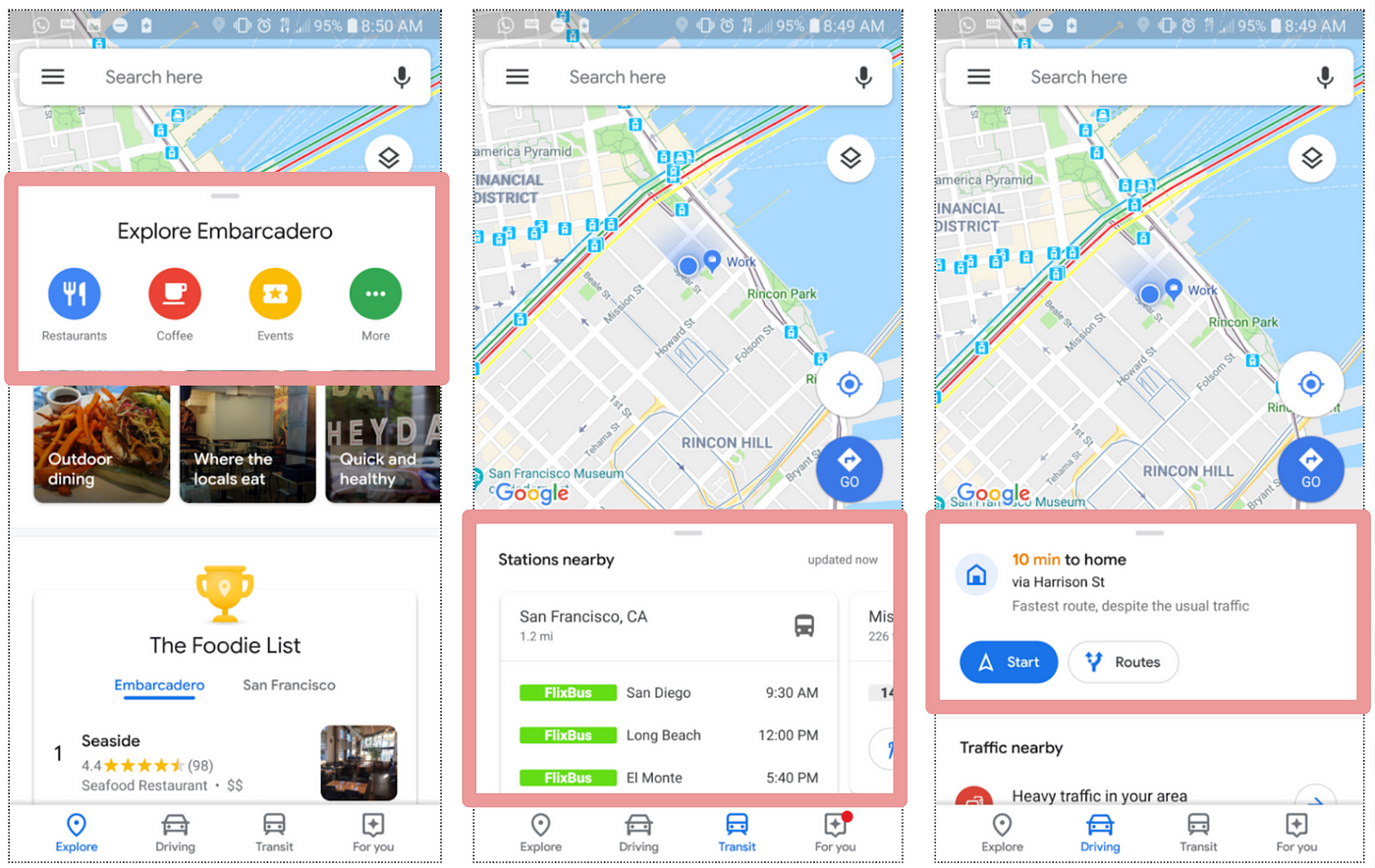The image contains three detailed screenshots from a cellphone map application, each providing different functionalities and information related to San Francisco and the Embarcadero area.

1. **Left Screenshot: "Explore Embarcadero"**:
    - The leftmost screenshot features a pop-up window in the center, titled "Explore Embarcadero."
    - Below the title, there are four colored buttons: 
        - A blue button labeled "Restaurants."
        - A red button labeled "Coffee."
        - A yellow button labeled "Events."
        - A green button labeled "More."
    - Under these buttons, there is a section called "The Foodie List," marked with a small gold trophy icon, listing "Seaside" as a highlighted restaurant. 
    - The screenshot provides additional context, indicating that Embarcadero is a location in San Francisco, California.

2. **Center Screenshot: "Stations Nearby"**:
    - The central screenshot displays a highlighted area with a pink square, labeled "Stations Nearby."
    - This section provides specific stations and transport options:
        - "San Francisco, California, 1.2 miles."
        - Several FlixBus routes to destinations like San Diego, Long Beach, and El Monterey, labeled "Corral Monte."

3. **Right Screenshot: "10 Minutes to Home via Harrison Street"**:
    - The rightmost screenshot highlights a boxed area in pink, informing the user that it takes "10 minutes to home via Harrison Street," despite unusual traffic.
    - It features a blue "Start" button for initiating navigation and a secondary button labeled "Routes" for alternative paths.
    - Each screenshot includes a map view in the upper portion, showing the geographical layout of the San Francisco or Embarcadero area.

The overall image vividly elucidates the rich functionalities of the map application, ranging from exploring local amenities and restaurant recommendations to providing real-time transit options and efficient navigation routes in San Francisco's Embarcadero area.